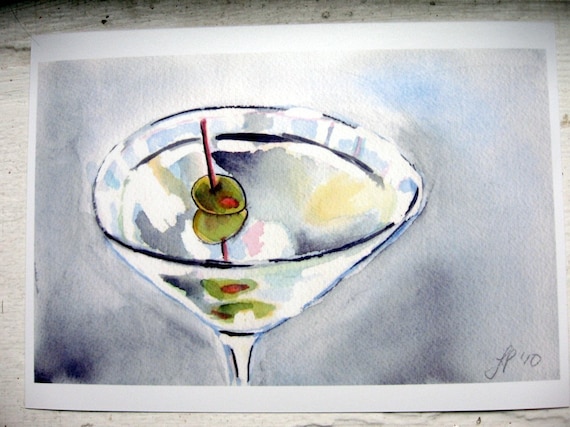This is a photograph of a watercolor painting depicting a martini in a standard martini glass. The glass holds a clear liquid and is slightly off-center to the left on the white cardstock canvas. In the center of the drink, two green olives are skewered on a stick, which appears red. Reflections of the olives can be seen both on the surface of the martini and through the glass, creating an illusion of having four olives. The vibrant green of the olives stands out as the brightest element in the painting, followed by subtle watercolor elements of black, yellow, light pinks, and blues. The background features a light, watercolor wash of black and white with touches of light blue, predominantly towards the top right corner, and darkens toward the bottom. The glass appears non-uniform, slightly wider on the right side, adding a unique character. At the bottom right corner of the painting are the artist’s initials "F.P." followed by the number "10."